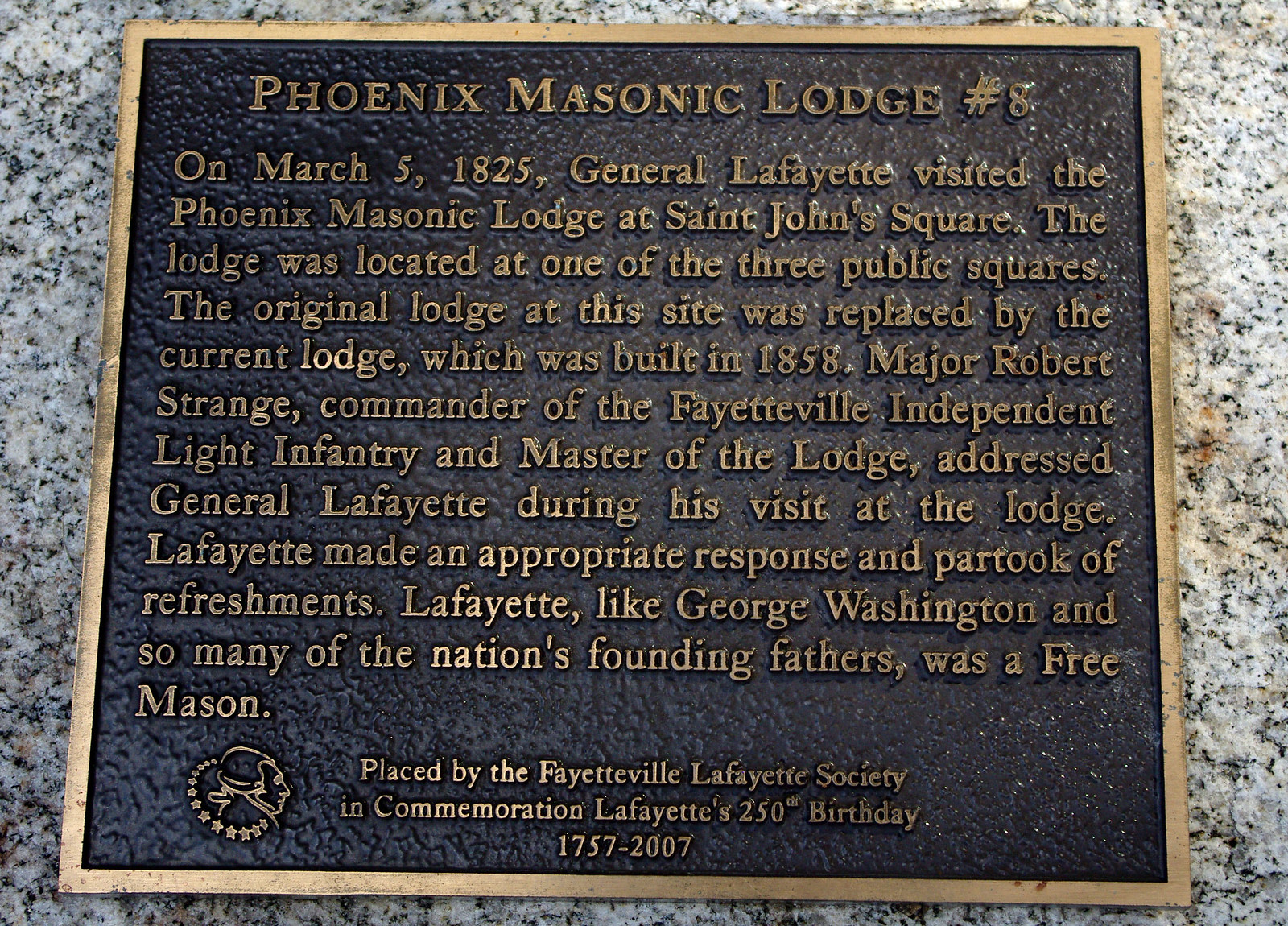This image captures a commemorative plaque made of brass, mounted on a marble-like background within an interior setting. The plaque is outlined with a distinctive golden frame, with the text inscribed in matching golden letters against a black backdrop. The heading reads "Phoenix Masonic Lodge #8." It details a significant historical event: General Lafayette's visit to the Phoenix Masonic Lodge at St. John's Square on March 5, 1825. This lodge, originally located at one of the three public squares, was replaced by the current structure erected in 1858. During Lafayette's visit, Major Robert Strange, commander of the Fayetteville Independent Light Infantry and master of the lodge, addressed him. Lafayette responded graciously and partook of refreshments. Like George Washington and many other founding fathers, Lafayette was a Freemason. This plaque, which features a logo depicting a face and stars in the bottom left corner, was placed by the Fayetteville Lafayette Society in 2007 to commemorate the 250th anniversary of Lafayette's birth, from 1757 to 2007.